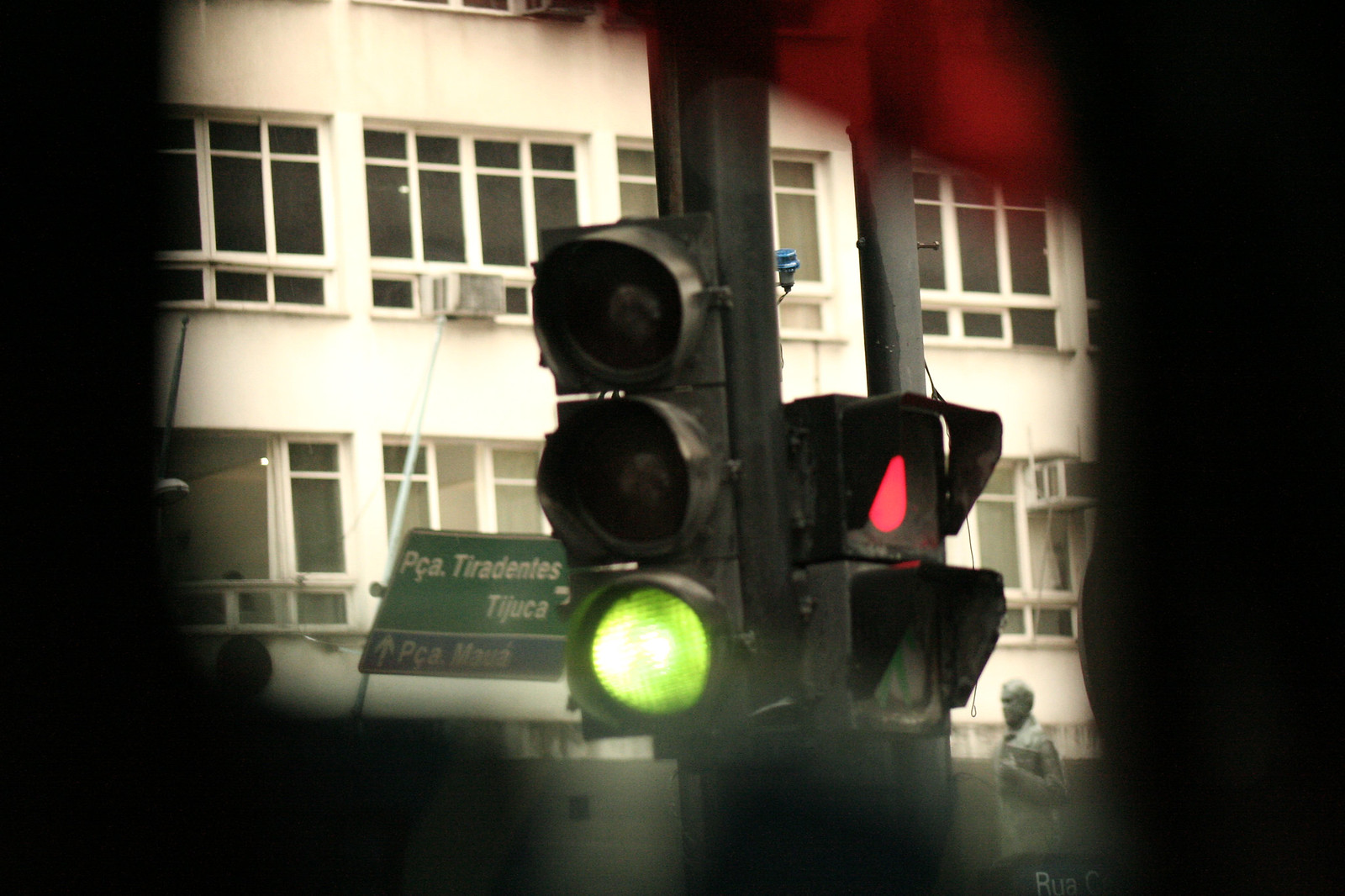The photograph, seemingly taken through a small, irregularly shaped opening in a dark space, captures an urban street scene. The central focus is a traffic light on a black post with the green light illuminated. To the right of it, there is a pedestrian signal displaying a red light. In the background, a large white building with numerous black-edged windows dominates the scene, some of which have air conditioners installed. A green directional street sign with white lettering, possibly in Portuguese or Spanish, is visible to the left of the traffic light. In the lower right corner of the image, a man walks down the sidewalk carrying a book against his chest. The edges of the photograph are framed in darkness, highlighting the view through the confined opening.